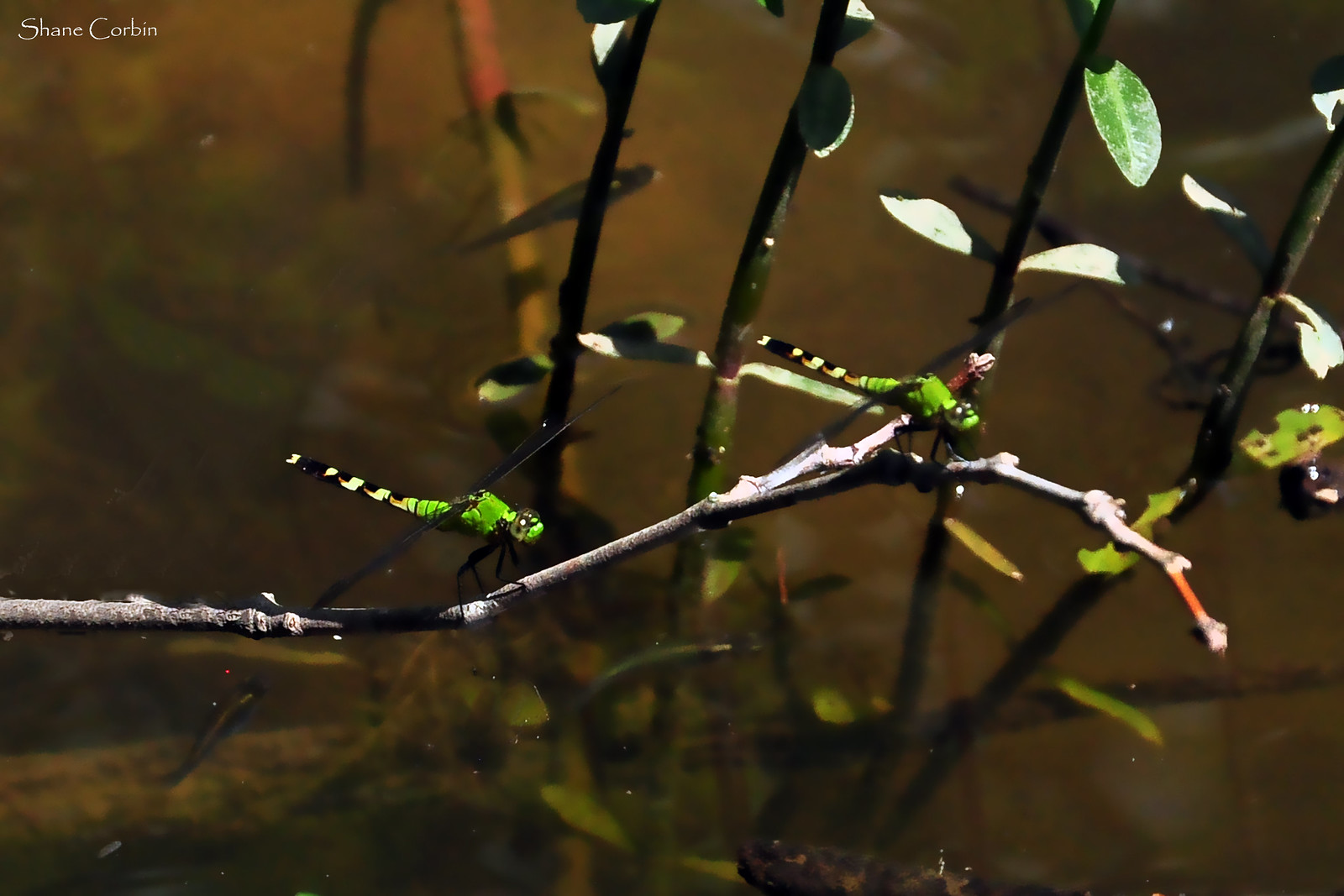In this close-up image, we see two bright lime green dragonflies perched on a single twig that extends from the left-hand side of the frame. The dragonflies take center stage in the composition, their bodies angled slightly to the right. Each dragonfly has black, white, and orange-ish striped tails and delicate, narrow wings that are faintly visible and dark in color. The twig from which the dragonflies rest emerges and curves upwards slightly before dipping at the end. 

The background features a blurred, murky swamp-like scene with four additional vertical stems adorned with leaves, giving the impression of a dense and overgrown environment. Elements such as limbs and leaves are discernible in the murky water below, adding to the natural, wild atmosphere of the photograph. In the upper left-hand corner, the photographer's name, Shane Corbin, is displayed in white text.